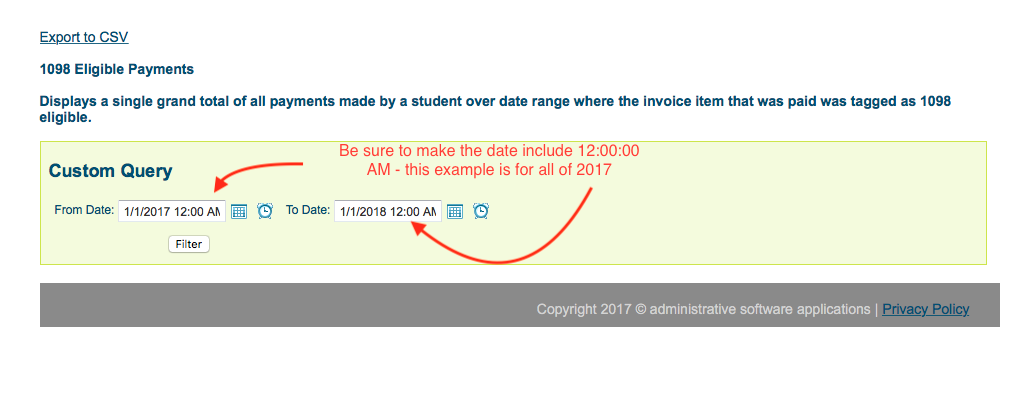Caption: 
"Export eligible payments to CSV: This feature allows administrators to export a detailed list of all payments made by a student over a specified date range, where each invoice item paid is tagged as 1098 eligible. The system displays a single grand total of these payments. In this example, the custom query covers the entire year of 2017, from January 1, 2017, 12:00 AM to January 1, 2018, 12:00 AM. The interface is set against a yellow background, and the filter is specified for administrative software applications from the year 2017. Privacy policy terms are also included."